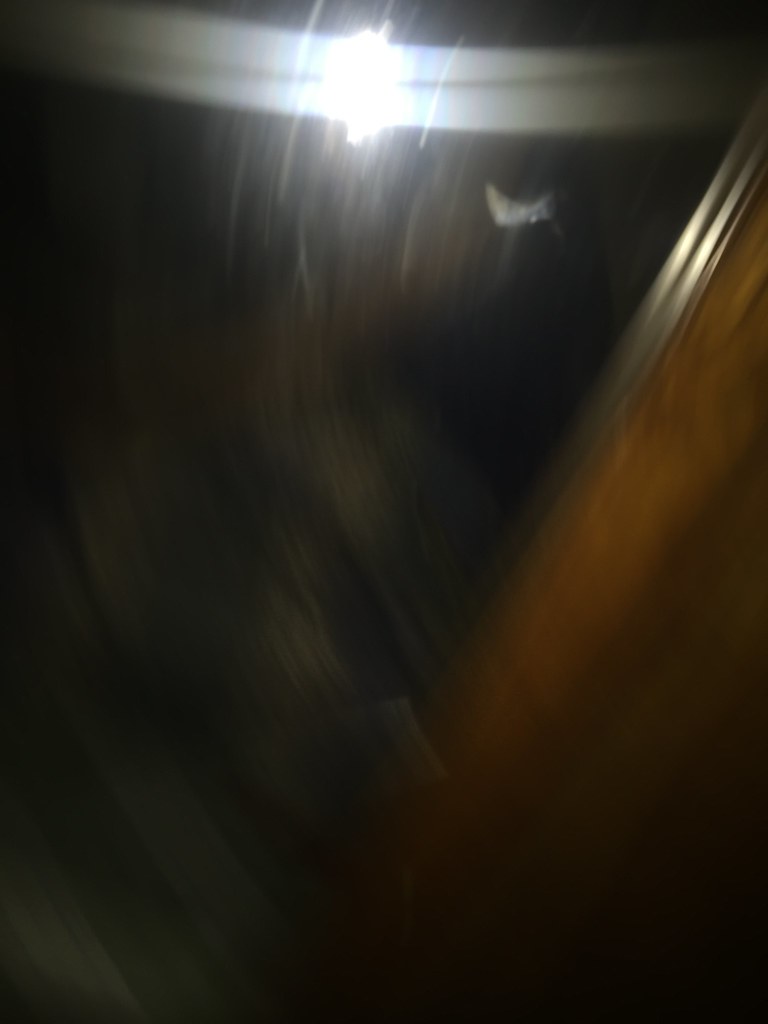The image is a vertical rectangle with the longer dimension running from top to bottom. It appears blurry, adding an element of mystery and making it somewhat challenging to discern specific details. At the very top center, there is a bright light, possibly mounted on a white horizontal post that spans from the left edge to the right edge of the image. Descending diagonally from the top right towards the middle bottom, there is a brown wooden post or door frame, tilted and cutting across the scene. In the upper right of the picture, there seems to be a small object in motion, potentially a bug, caught mid-flight. The image likely captures a nighttime scene, evident by the predominantly black background. Additionally, there are indistinct, blurred lines around the bright light and curving around the bottom left corner, perhaps indicating motion or an artifact of the camera's exposure.